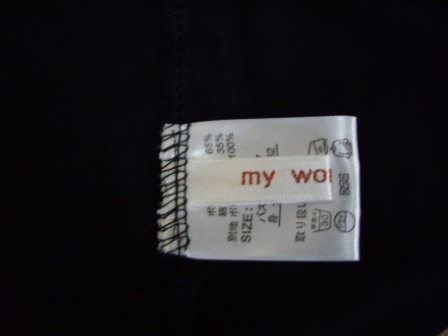The image displays two tags attached to a black piece of clothing, set against a black background in a square-shaped frame. The upper tag is smaller and rectangular, white in color with "MYWO" written in red text. Below it, there's a larger, square-shaped care tag, which is also white. This lower tag features black text and artwork, including the word "SIZE" in the top left corner along with the fabric composition mentioned as "65% 35%." Additionally, there are black symbols indicating washing instructions, potentially including Japanese characters. The tags are sewn onto the black fabric with black threads, suggesting they're care labels for the garment. For accurate viewing, the image might need to be rotated once to the right.